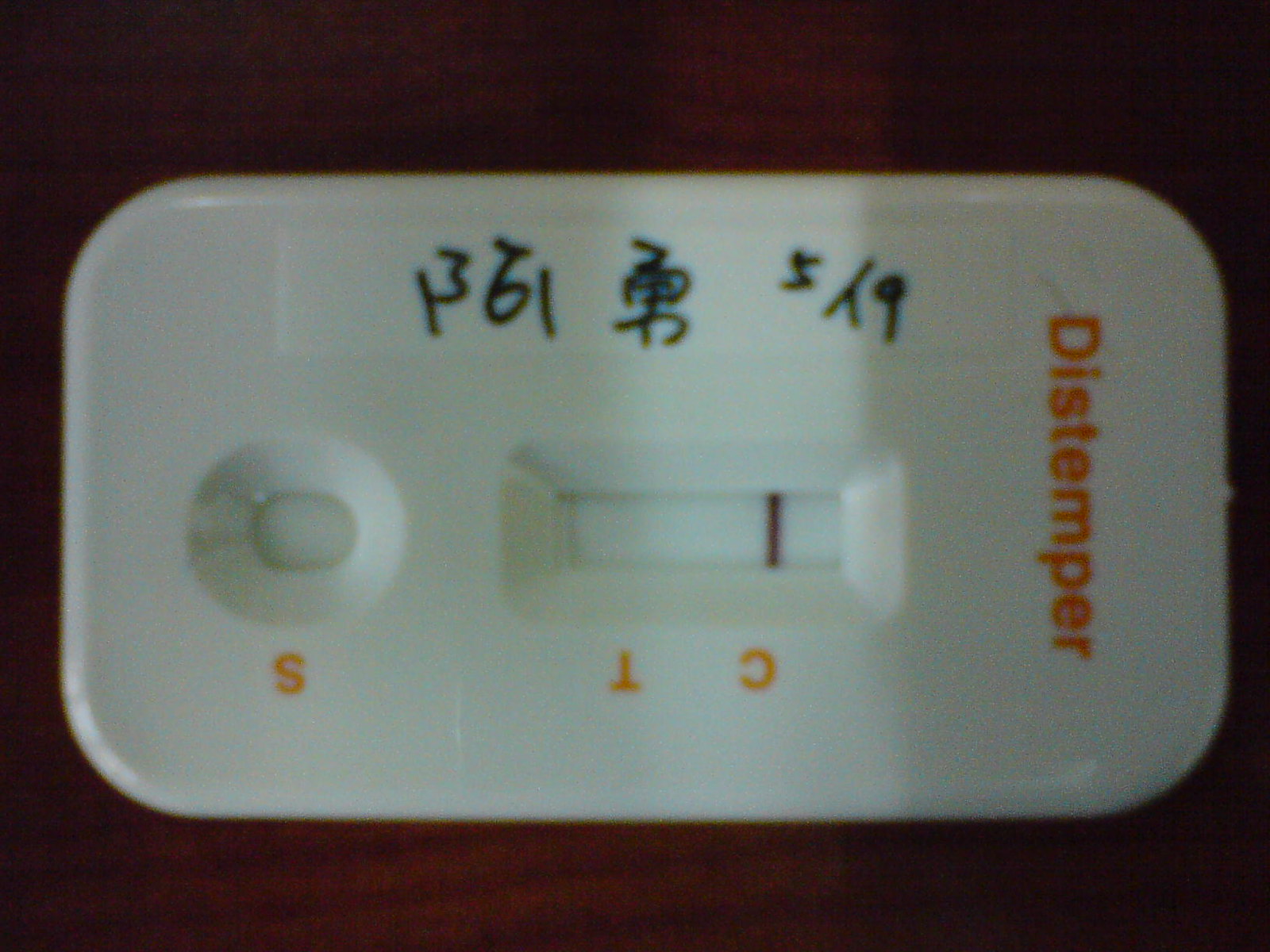The image displays a close-up view of a medical testing device, prominently occupying approximately 75% of the frame. The device, characterized by its rectangular shape with rounded corners, is set against a flat, darker walnut wood background, featuring a subtle grain texture.

The device itself is white and features what appears to be Chinese or Japanese writing at the top. Notably, at the very top in orange text, the word "distemper" is visible. Central to the device is a window marked with the letters “C” and “T” in orange, with a dark line visible next to the "C," indicating a test result. At the bottom of the device, there is a circular indentation marked with an "S," likely intended for depositing a fluid sample such as blood or saliva.

The image is slightly out of focus, lending a blurred quality to the details. The right side of the device shows signs of shading, contrasting with the lighter appearance of the left side. The overall composition emphasizes the device's functional aspects against its organic wood background.